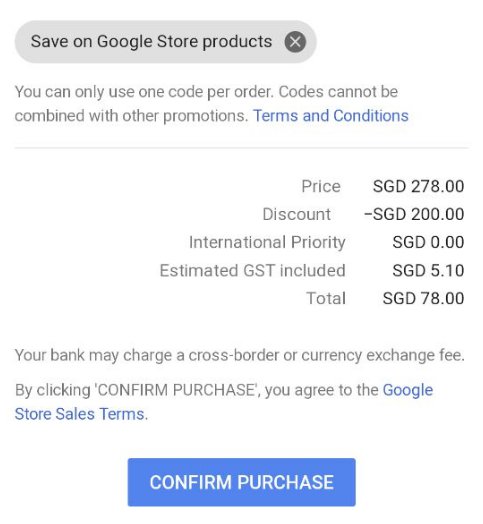The image features a grayish bubble in the upper left-hand corner, extending slightly past the center towards the right side. Inside the bubble, there is a light gray background with the text "Save on Google Store products" written in black font. Within the gray bubble, on the left side, there is a small gray circle with a white ‘X’ symbol, functioning as a close button.

Below this section, there is black text stating, "You can only use one code per order. Codes cannot be combined with other promotions." The phrase "terms and conditions" follows this statement in blue font, indicating that it is a clickable hyperlink.

Separated by a thin gray line, the next section of the image contains right-justified information related to an order summary:

- Price: SGD 278
- Discount: minus SGD 200
- International priority: SGD (amount not specified)
- Estimated GST included: SGD 5.10
- Total: SGD 78